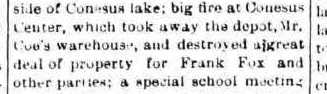The image features a vintage black-and-white newspaper column, centered against a stark white background. The snippet is narrow and horizontally oriented, consisting of five lines of text with a thin vertical rule on each side. The text, rendered in black, includes the phrases: "Side of Consensus Lake, Big Tire at Kinesis Center, which took away the depot, Mr. Ko's Warehouse, and destroyed a great deal of property for Frank Fox and other parties, a special school meeting." Adjacent text from another column to the right is partially cut off. The overall appearance suggests a small, aged cutout from a historical newspaper, surrounded by a completely white backdrop which emphasizes its antiquated style and content.